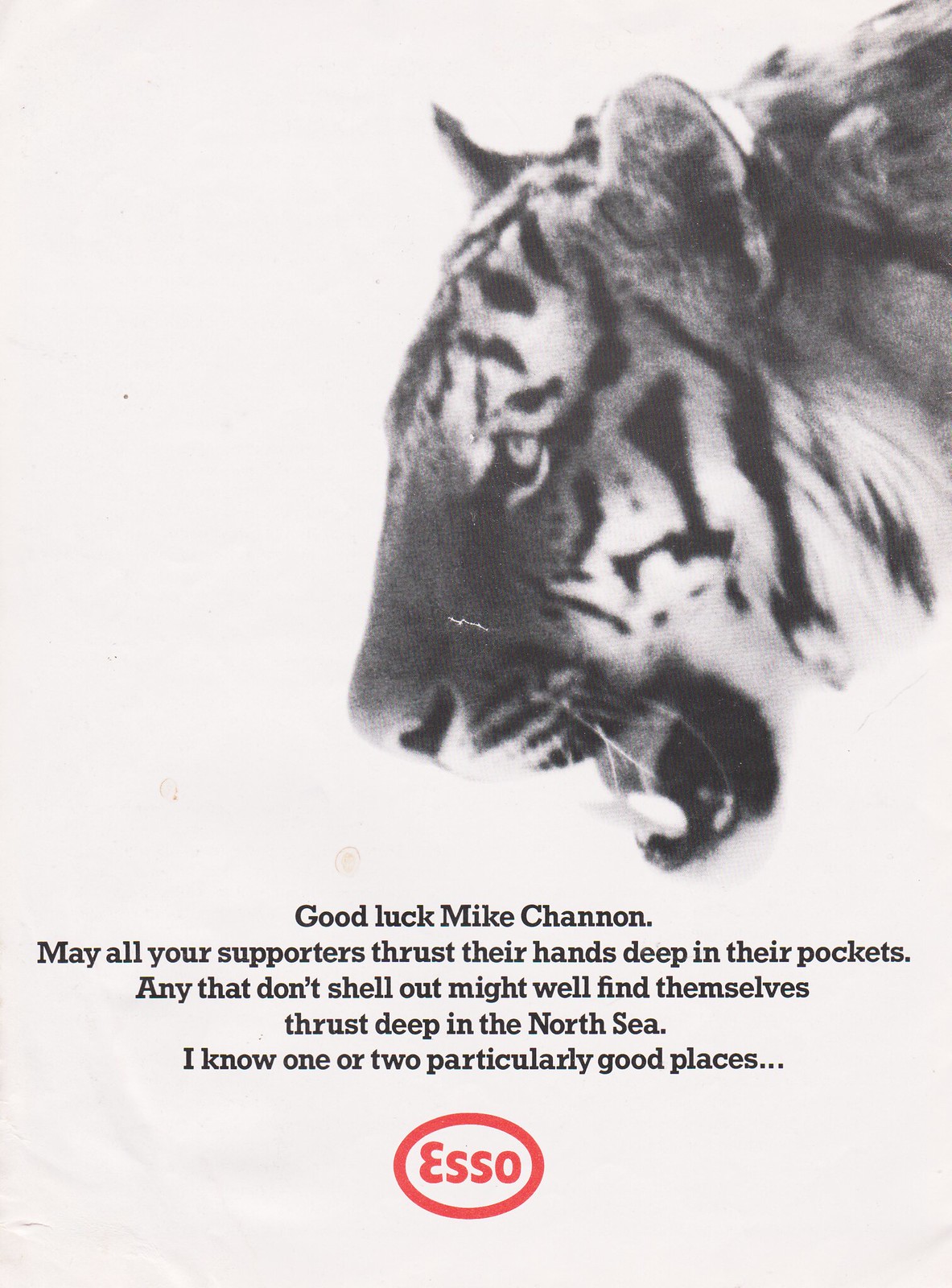The image appears to be a poster featuring a prominently displayed, black-and-white photo of a tiger's head in the upper right corner. The tiger looks menacing with its head angled down, mouth open to reveal sharp teeth, and eyes looking to the left, against a stark white background. Centered below the tiger's face is a block of black text that reads: "Good luck, Mike Shannon. May all your supporters thrust their hands deep in their pockets. Any that don't shell out might well find themselves thrust deep in the North Sea. I know one or two particularly good places." At the bottom of the image is a red-outlined oval with the word "ESSO" in red letters inside it, positioned against the white background. The overall tone of the poster suggests a message of farewell or good wishes, possibly for someone retiring.